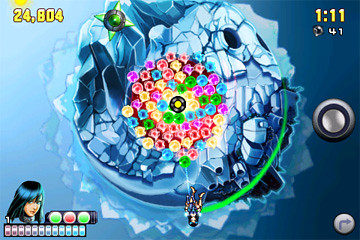The image is a vibrant screen capture from a mobile video game, showcasing an animated, colorful scene. Centrally, a large spherical, planet-like object predominantly displays a mix of brightly colored gems, including green, blue, red, pink, purple, and yellow, all concentrated within a circular arrangement. At the very core of this sphere sits a black, doughnut-shaped feature. The background of the image transitions from a lighter blue on the left to a darker blue on the right, resembling an icy or watery planet. Below the large object stands an upside-down female cartoon character with long, dark hair, positioned as if on the South Pole, possibly holding a rope connected to the sphere. The character appears near several numerical and graphical elements: the top left corner shows a score of 24,804 in yellow, the upper right corner includes a timer showing 1:11, and below it, an emblem marked with 41. The bottom left corner features an image of a girl’s face with long, dark hair next to an indicator resembling a stoplight with two green dots and one red dot. Additionally, a gray, stainless steel-like button and a right-turn arrow are present near the top center-right, accompanied by a green streak encircling the main sphere, all contributing to the dynamic and engaging interface of the game.